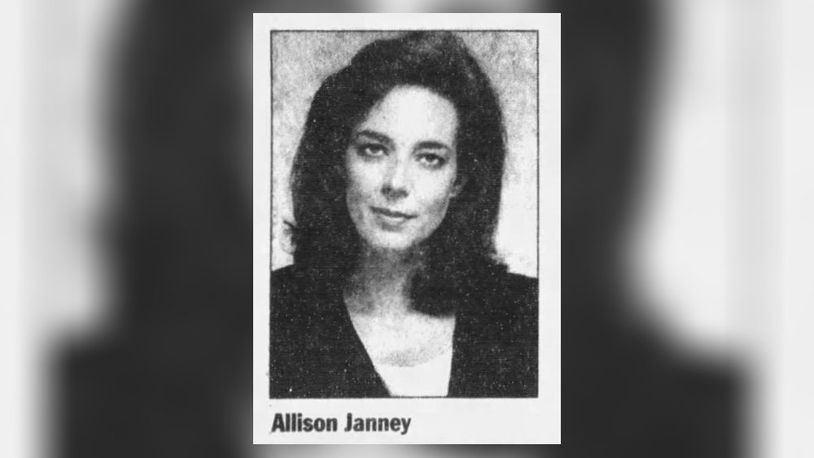This image is a black-and-white photograph of a woman named Allison Janney. The photo has an old, vintage style with significant noise and is centered within a white rectangular frame. Behind this framed photo is a larger, blurred version of the same image, serving as the background. In the bottom left-hand corner of the photo, the name "Allison Janney" is printed in black text. The woman, who is looking slightly upwards, has medium-length, dark hair that falls to her shoulders. She is not wearing any jewelry and is dressed in a dark outfit, possibly a black dress with a plunging neckline. The overall composition and layout suggest it could be an ID card or a yearbook photograph, with her likeness in a somber, straightforward pose.